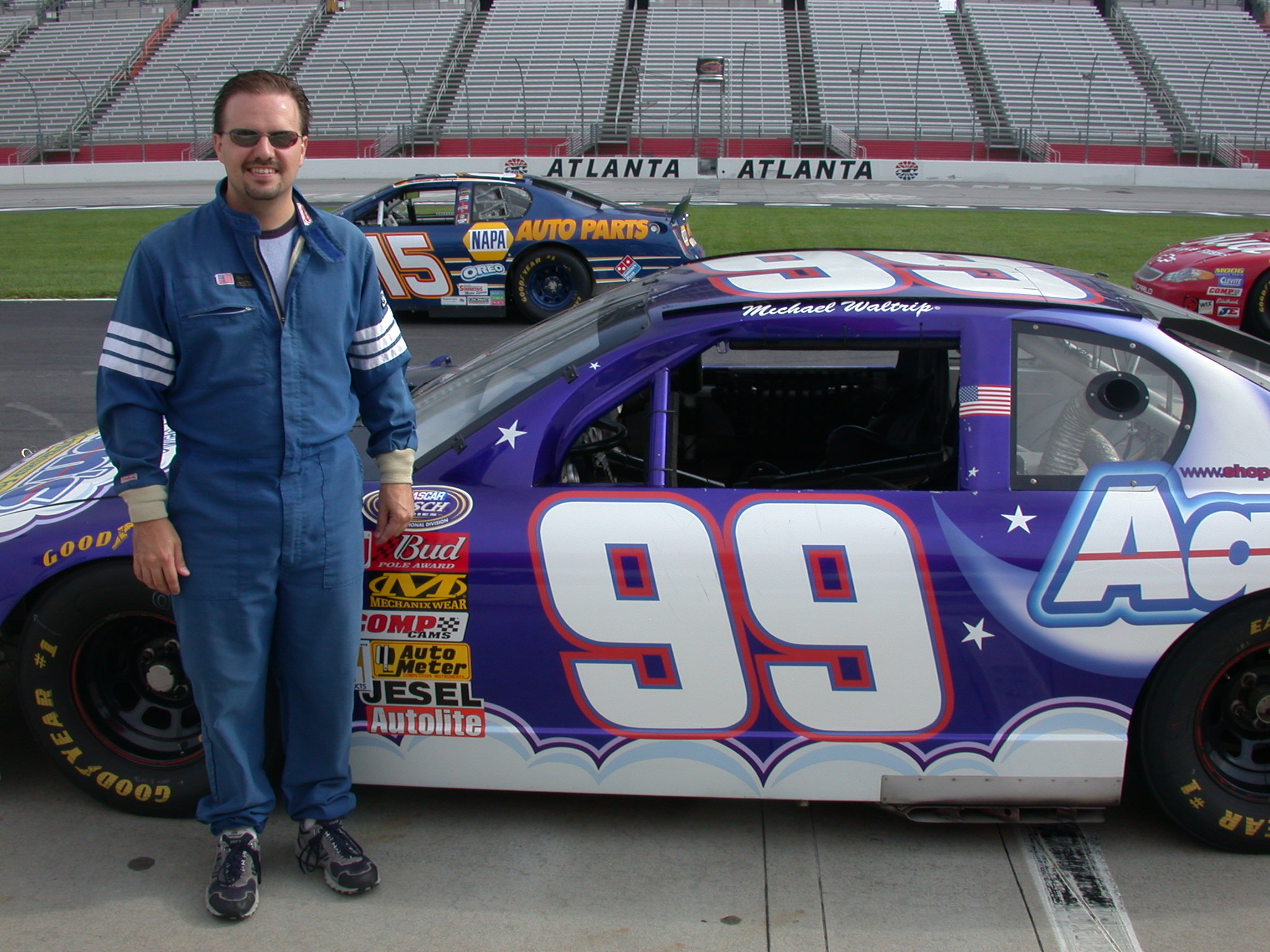In this vividly detailed photograph taken outdoors at a racetrack, a race car numbered 99 takes center stage. The car, painted in a captivating blend of dark blue and purple hues adorned with a celestial design featuring a moon, stars, and clouds, is strategically positioned in front of the stadium bleachers with "Atlanta Atlanta" visibly inscribed in the background. The car boasts an array of sponsor decals from prominent names such as Bud, Busch, M, Comp, Auto Meter, Jesel, and Autolite, with the Goodyear-branded tires accentuating its racing pedigree. Notably, the number 99 is boldly displayed in white font on both the side and the roof of the car, and just above the door frame, the name "Michael Waltrip" is clearly readable.

In the foreground, standing next to the car, is the race car driver clad in a striking blue jumpsuit accented with white stripes on the arms. He sports slicked-back dark brown hair, a mustache, beard, and is equipped with stylish sunglasses and sneakers. His composed stance partly obscures the front of the car, particularly the hood, and he is located to the left of the vehicle. The scene is further enriched by the presence of additional race cars in the background, including a notable dark blue car marked with the number 15.